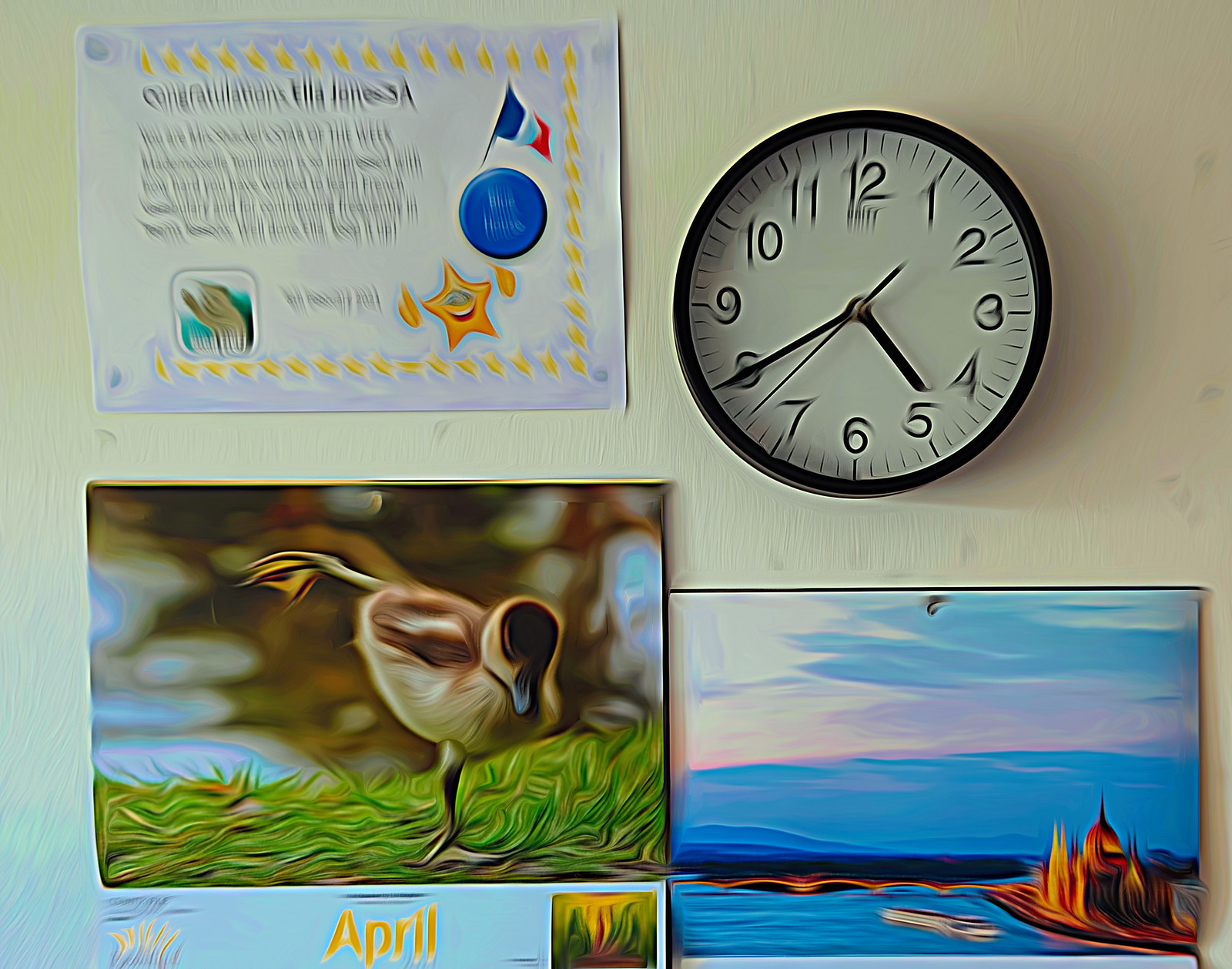This surrealist digital artwork captures a classroom wall adorned with various heavily blurred elements. The background is a beige, painted wall that supports a visually incoherent assemblage of objects arranged in a rough square formation. The upper left corner features a stretched and distorted certificate with an indistinct star and a French flag; the vague text seemingly congratulates someone named Ella Jones. Below this certificate is an enigmatic painting of a duckling, posed with one leg lifted, which also suggests it might be a calendar due to the discernible word "April" beneath it. Directly adjacent to the certificate and near the top right is an analog clock with smeared, stretched numbers, indicating the time as 4:40. Beneath the clock lies a surreal landscape painting depicting a ship near an Indian temple by the sea, surrounded by pink and blue skies. The entire composition appears to be purposefully blurred, evoking a surrealistic and dreamlike atmosphere achieved through digital manipulation.